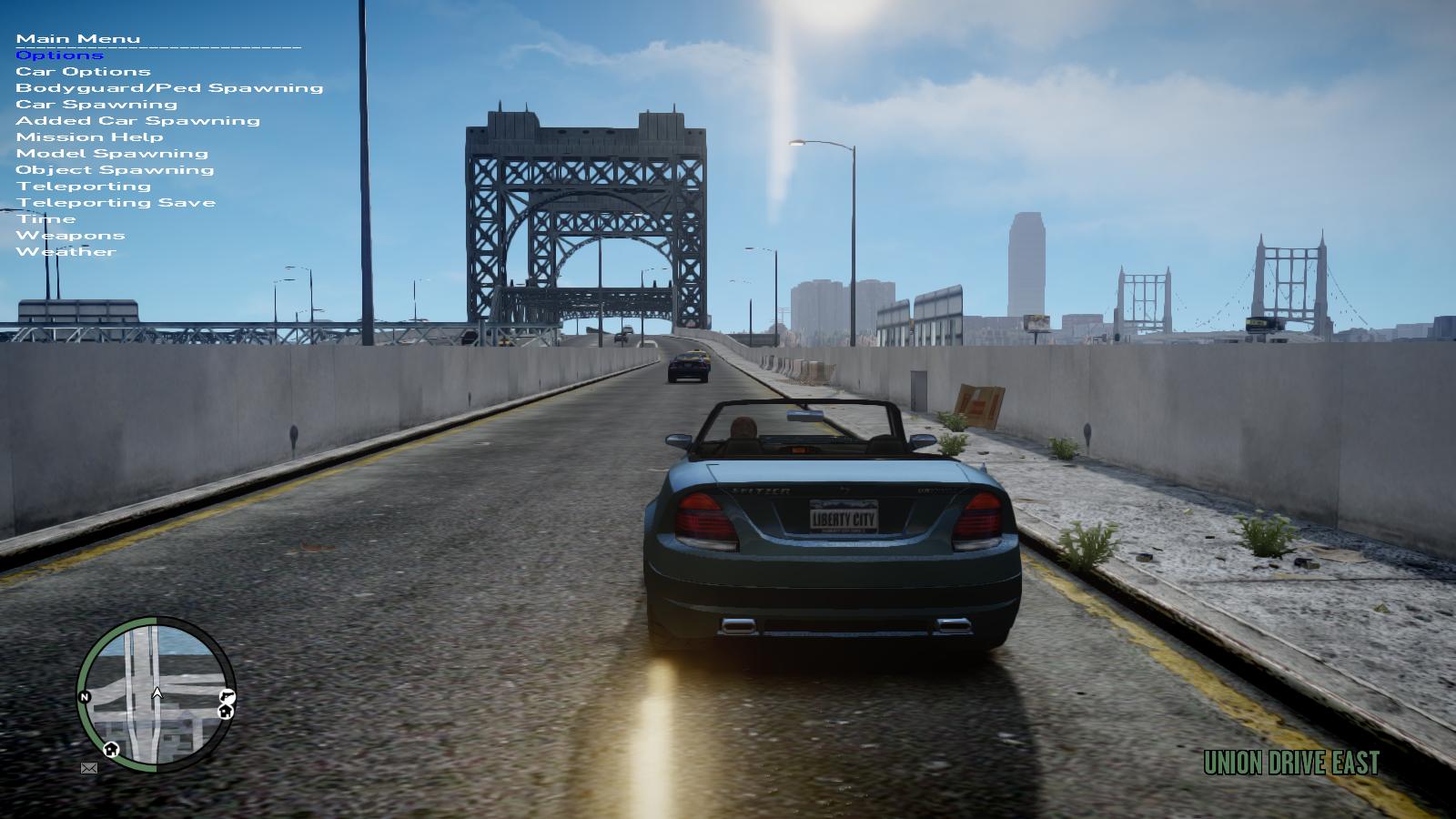This detailed image appears to be a screenshot from a video game, likely from Grand Theft Auto given the numerous indicators. The foreground features a light blue convertible with a Liberty City license plate, suggesting it might be from GTA 3. The driver inside the vehicle has short hair, although their gender is undetermined. The car is shown driving down a cement bridge under clear blue skies with a few clouds.

The bridge itself is defined by large concrete barricades on both sides, with tall light or telephone poles lining the right edge. Green archways with intricate patterns span the bridge, and in the distance, tall buildings can be seen silhouetted against the sky. A single car, indistinguishable in color, is driving ahead of the blue convertible.

On the bottom left corner is a minimap. The left border of the minimap is light green, likely indicating a health bar, while the right side is black. The map displays various roads similar to those seen on Google Maps, and includes small icons, one with an 'N' denoting North. Green text at the bottom right reads "Union Drive East."

In the upper left corner, the game interface has a white text menu titled "Main Menu," followed by "Options" in blue text, and several other items in white text. These menu options are listed vertically and include: Car Options, Bodyguard/PED Spawning, Car Spawning, Added Car Spawning, Mission Help, Model Spawning, Object Spawning, Teleporting, Save, Time, Weapons, and Weather. This comprehensive menu suggests the image may be from a modded or debug version of the game.